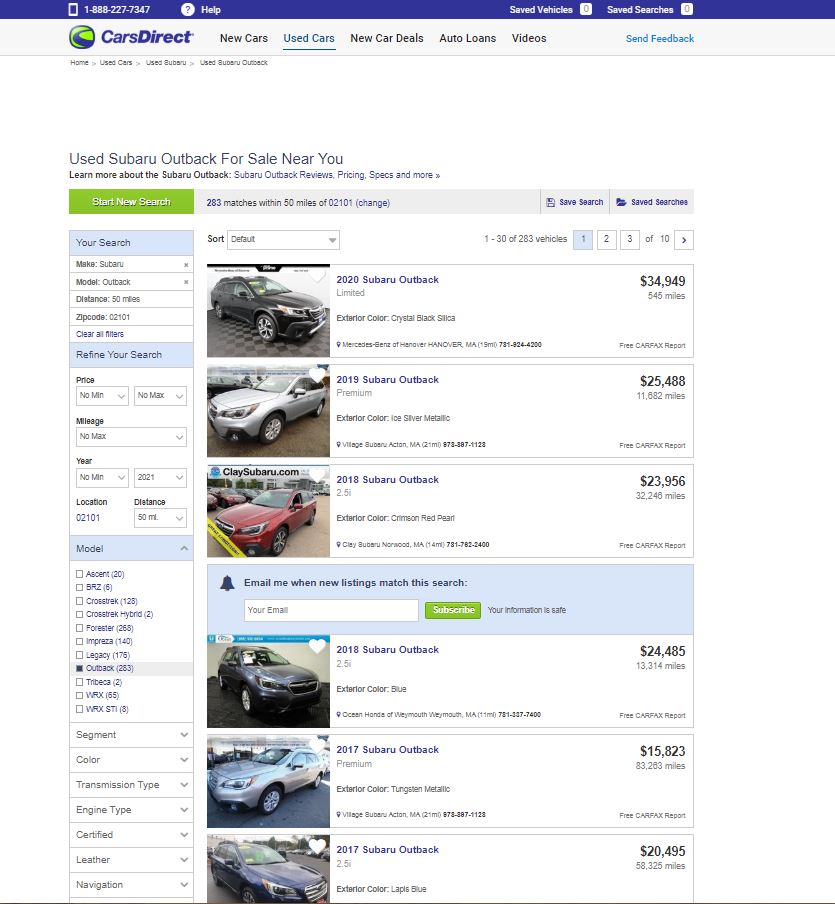A detailed screenshot captured on a desktop or laptop computer shows the Cars Direct website interface. At the top, there is a prominent purple banner featuring the contact number 1-888-227-7347, accompanied by accessible icons for Help, Saved Vehicles, and Saved Search. Directly below this banner, on the bottom left, sits the Cars Direct logo alongside a green logo depicting a purple road.

In the website's navigation bar, users can explore options including New Cars, Used Cars, New Car Deals, Auto Loans, and Videos. To the far right of this bar is a 'Send Feedback' button. The focus of the user's current search is for a used Subaru Outback available for purchase in their vicinity.

Starting a new search reveals that there are 283 Subaru Outback matches within a 50-mile radius of the zip code 02-101. The search results showcase various models including a 2020 Subaru Outback listed at $34,949, a 2019 Subaru Outback at $25,488, a 2018 Subaru Outback available for $23,956, another 2018 Subaru Outback priced at $24,485, a 2017 Subaru Outback for $15,823, and another 2017 model for $20,495. These vehicles display a range of colors including black, silver, red, and blue, with all of them having an approximate mileage of 50,000 miles.